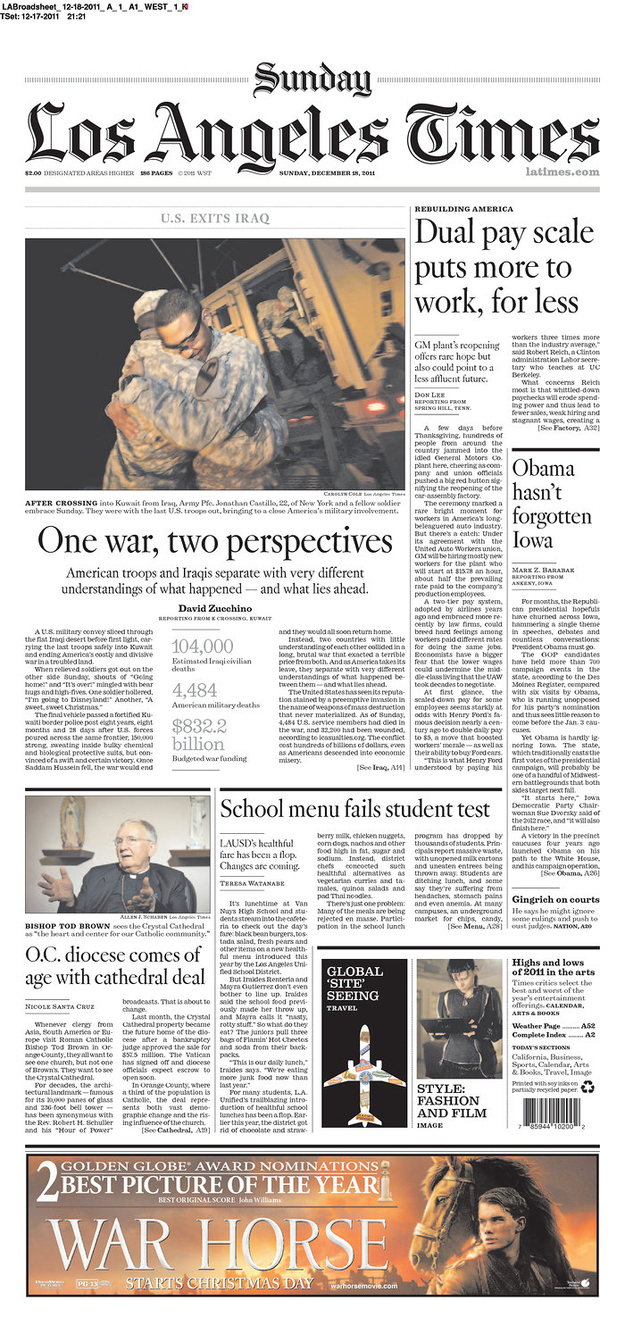Category: Websites

Caption: The image showcases the front page of the Los Angeles Times newspaper. The headline reads "Sunday, Los Angeles Times, $2, Sunday, December 18, 2011" and the website URL "latimes.com" is also displayed. The main headline, "US Exits Iraq," is accompanied by a photo of two military personnel hugging each other, symbolizing the emotional conclusion of the war. The accompanying article is titled "One War, Two Perspectives," offering insights into the departure of American troops from Iraq. Another prominent headline reads "Rebuilding America: GM Plants Reopening Offers Rare Hope but Also Could Point to a Less Affluent Future," discussing the revival of General Motors plants. Additionally, the front page features stories such as "Obama Hasn't Forgotten Iowa" and "School Menu Fails Student Test." The final headline reads "OC Diocese Comes of Age with Cathedral Deal," emphasizing significant local developments.